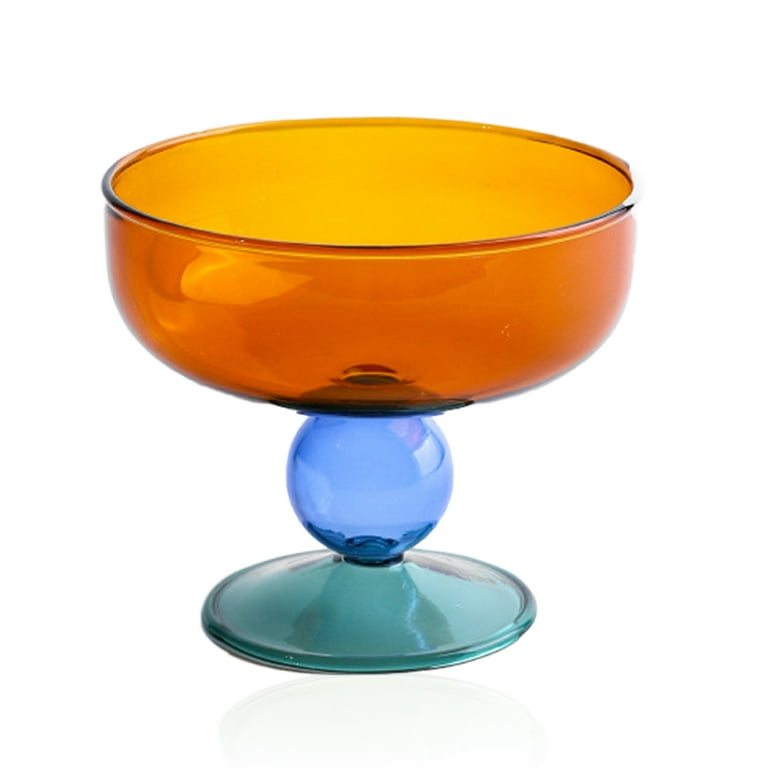The image displays a decorative glass sculpture composed of three distinct sections, all resting on a white background. At the bottom is a clear light blue glass base, measuring approximately four inches in diameter. Attached to this base is a round orb made of darker blue glass, maintaining its translucent quality. The top section features a wider, bowl-shaped glass element, constructed from light orange, see-through glass. This bowl is about six inches in diameter and stands three to four inches high, slightly taller than the blue orb beneath it. The entire sculpture is seamlessly fused together, highlighting an artistic style that emphasizes transparency and color gradation, making it suitable for both decorative and functional uses.